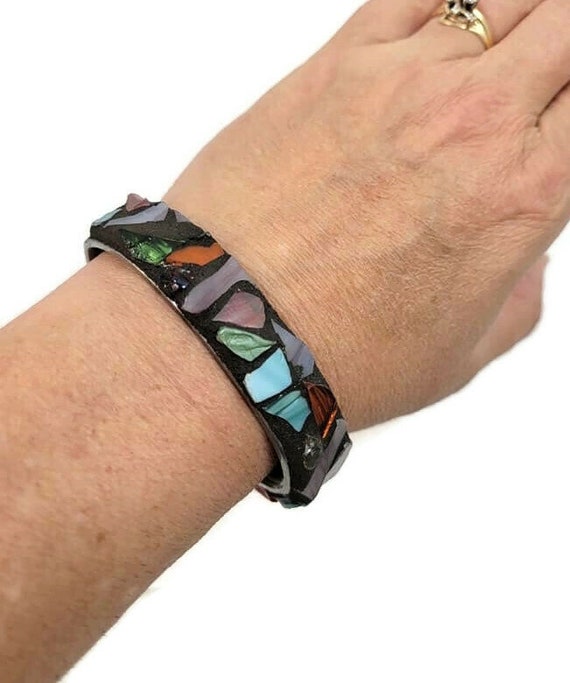This detailed photograph showcases the outstretched left arm, wrist, and partially visible hand of a light-skinned person, likely a woman, adorned with distinctive jewelry. The focus is on a striking bracelet encircling the wrist, characterized by a predominantly black background and an artisanal appearance. This bracelet seems crafted from a combination of black resin over a metal base and is inlaid with an array of colorful stones or perhaps intricate plastic or resin pieces. These embedded elements are of various shapes and sizes—ranging from circular and rectangular to jagged pieces, suggesting a handmade, eclectic design. The stones showcase a spectrum of colors, including vibrant green, purple, blue, red, orange, and even onyx-like black, creating a vivid, mosaic-like pattern. Accompanying this bracelet is a gold ring on the ring finger—possibly a wedding ring with a small, noticeable stone, adding elegance to the overall appearance. The visible skin appears somewhat dry, accentuating the natural, unpolished aesthetic that harmonizes with the bracelet's rustic charm.